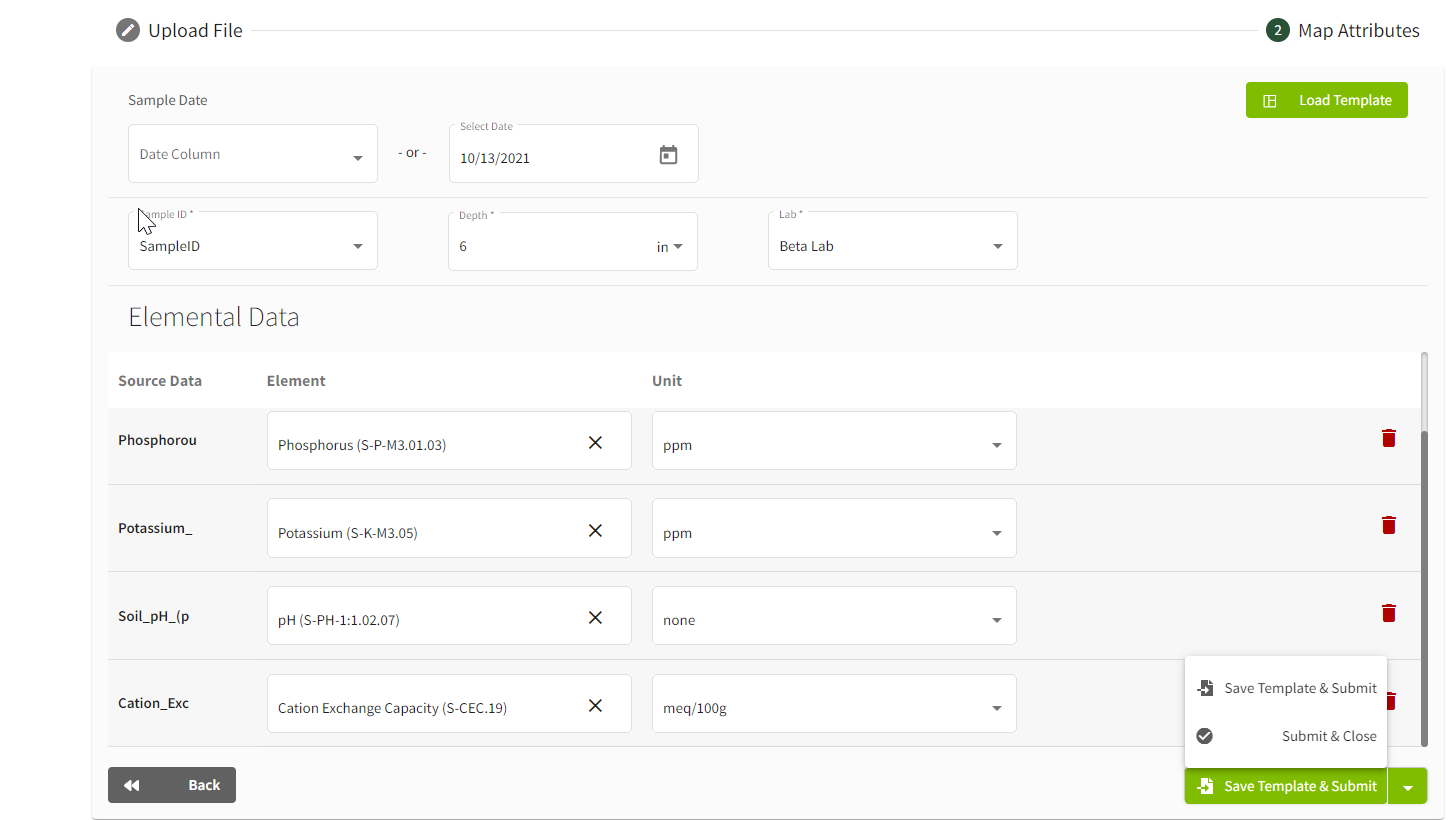The screenshot depicts a webpage interface primarily centered on file upload and mapping attributes. 

At the top of the page, the background is white. On the left, there is a small gray circle slightly overlapping the edge, containing a white pencil icon. Next to this circle, in gray text, are the words "Upload File," both starting with capital letters.

Moving to the right, a small dark green circle with the number "2" in white text is visible. Beside this circle, the words "Map Attributes" are displayed, each word also starting with a capital letter.

Beneath this section is a light gray background that serves as the primary working area of the interface. Here, the heading "Sample Date" is prominently displayed. Below this heading, there are dropdown menus. The first dropdown is labeled "Date Column or Select Date" and is currently set to "10-13-2021."

Following this, another field labeled "Sample ID" is shown with the value "Sample ID." This is followed by "In Depth," which is populated with the number "6," and "IN DIM." Further down is the "Lab" field, displaying "Beta Lab" with an associated dropdown menu.

The section then details "Elemental Data," including "Source Data" and "Source Data Elements Unit." The respective fields are already populated with their related elements and units.

At the bottom of the interface, two buttons are displayed. On the left, a "Back" button with a left arrow icon, and on the right, a "Save Template and Submit" button are present, offering options to either return to the previous screen or save and submit the form respectively.